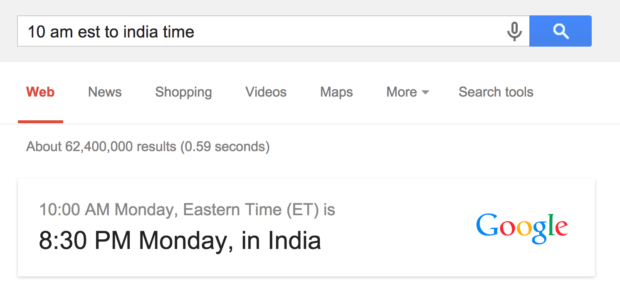This image depicts a screenshot set against a white background, showcasing a web page. At the top, there is a light gray header containing a search bar. Inside the search bar, black text reads "10 a.m. EST to India time." To the right of the search bar, a gray microphone icon and a blue magnifying glass icon are visible. 

Directly below the search bar, a horizontal menu features various options from left to right: "Web" highlighted in red text, followed by gray text options "News," "Shopping," "Videos," "Maps," and "More" which includes a pull-down arrow. Additionally, "Search tools" is written just below the menu.

In the lower right corner of the image, a large, colorful Google logo is present. To the left of this logo, the text "10 a.m. Monday Eastern Time (ET) is 8:30 p.m. Monday in India" is displayed, clarifying the time conversion from EST to India time.

This detailed depiction captures the essential elements of the screenshot, including the design of the search interface and the specific information about the time conversion.